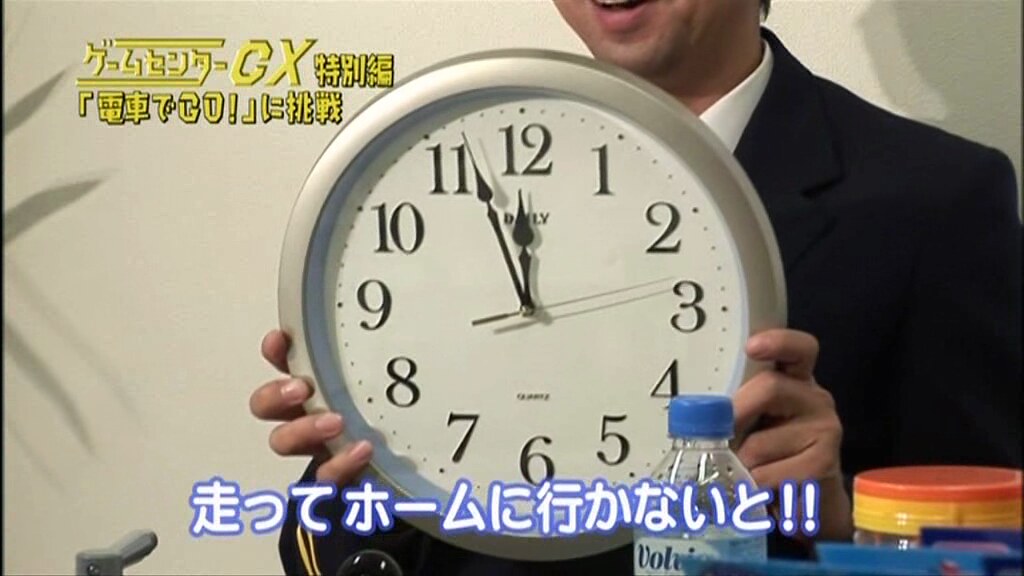In the image, a man dressed in a black suit with a white shirt is prominently holding a clock. The clock has a silver frame and features traditional numbering from 1 to 12. The hour hand points near the 12 mark, the longer minute hand is slightly past the 11, and the thin, silver second hand is positioned roughly halfway between the 2 and 3. The background showcases several elements, including Japanese writing and yellow text at the top left reading "CX." Additional Japanese text is visible at the bottom. Beside the man, there is a water bottle and another container with an orange top.